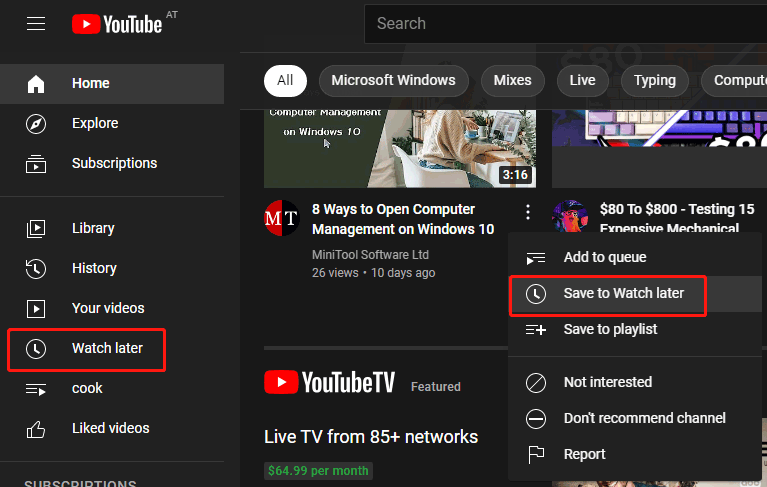This image is a screenshot of the YouTube homepage in dark mode, featuring a black background with white text. On the left side, the standard YouTube navigation column is visible, including tabs such as Home, Explorer, Subscribe, Library, History, Your Videos, Watch Later, and Liked Videos. Notably, the Watch Later tab is highlighted with a red rectangle.

In the main content area, there are one or two selected videos. One prominent video titled "Eight Ways to Open Computer Management on Windows 10" has a duration of 3:16 minutes. To the right of this video, the "Save to Watch Later" button is also highlighted with a red rectangle.

At the top of the screen, YouTube's standard category tabs are visible, which include All, Microsoft Windows, Mixed, Live, and Typing Computer, indicating the user's search context. 

Additionally, there is a YouTube TV advertisement at the bottom of the screen, promoting a live TV service with "85+ networks" for $64.99 per month. This screenshot illustrates a user saving a video to their watch later playlist.